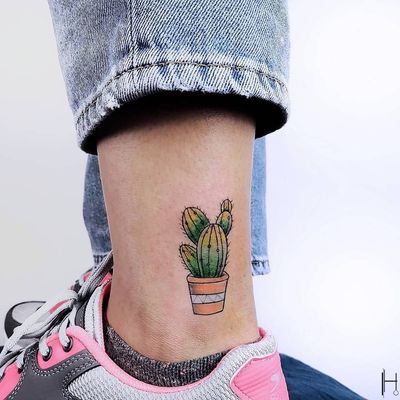This close-up image captures the ankle of a person, presumably a woman, showcasing a detailed and colorful tattoo. The tattoo features a green cactus growing in an orange terracotta pot adorned with a gray stripe. The individual is wearing pink athletic shoes with white and gray accents, alongside dark gray ankle socks. Her jeans, which are a faded blue, are intentionally pulled up on the left leg to display the tattoo fully, while the right leg's pant leg remains down. The background of the image is plain white, making the vibrant details of the tattoo and the pink sneakers more prominent. Additionally, there is a stylized "H" logo visible on the lower right side of the shoe, further emphasizing the attention to detail in this image.